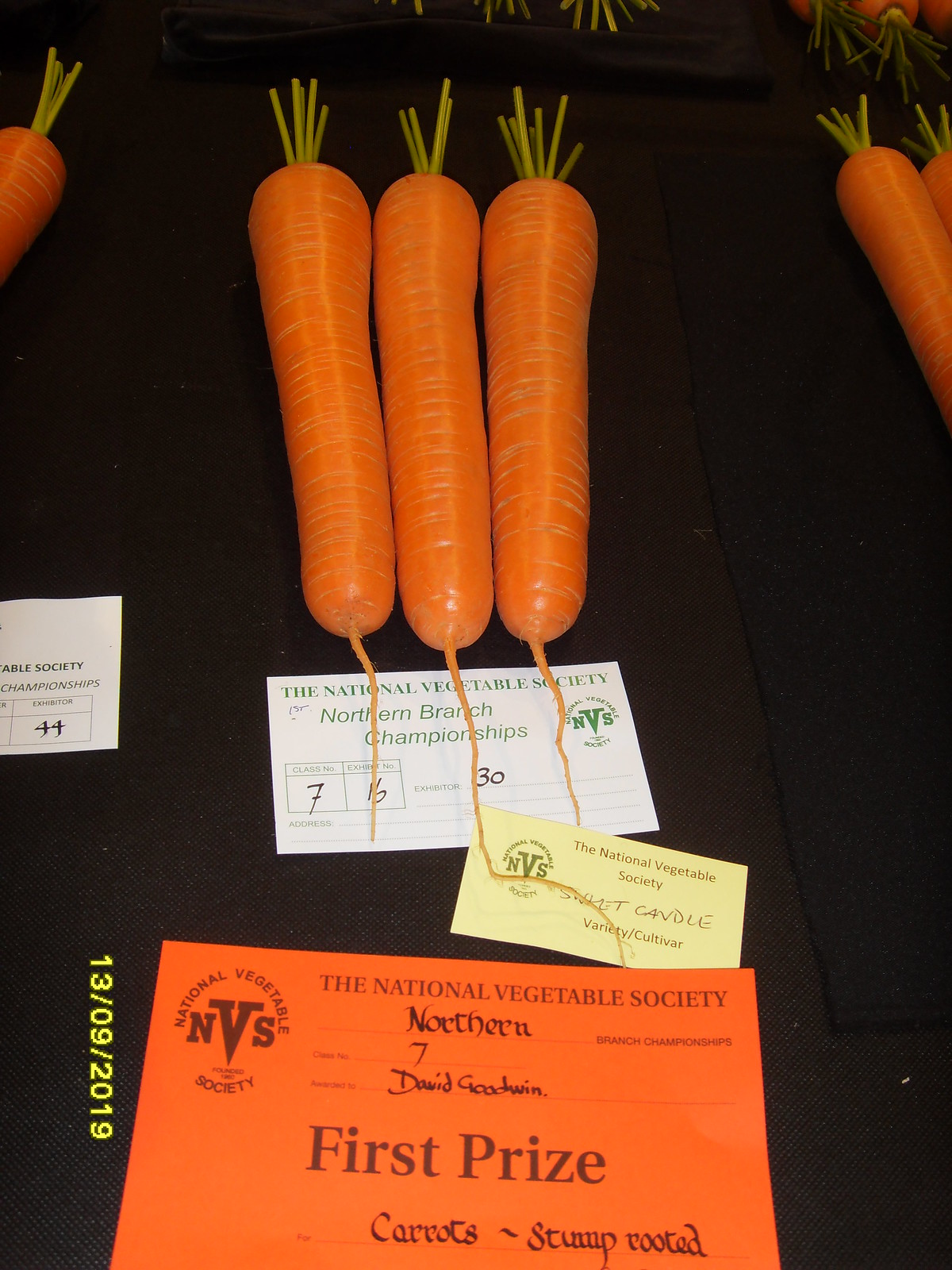In this vibrant full-color image, there are three bright orange carrots laid out on black felt, all identical in size, with symmetrical little green stems and smaller root offshoots protruding. They seem meticulously presented, suggesting their participation in a competition. To the left and right of the main trio, partially visible carrots imply a larger context, likely a farmer’s fair or agricultural event. 

Beneath the carrots, a series of documents and cards are visible, contributing to the narrative. A small white card under the carrots reads "National Vegetable Society Northern Branch Championships." Below it, an orange card with black text proclaims the carrots as having won first prize in the "stump rooted" category, awarded to David Goodwin. These accolades affirm the exceptional quality and presentation of the carrots, marking them as prize-winning specimens. The image is stamped with a date, 9-13-2019, situating this achievement at a specific point in time.